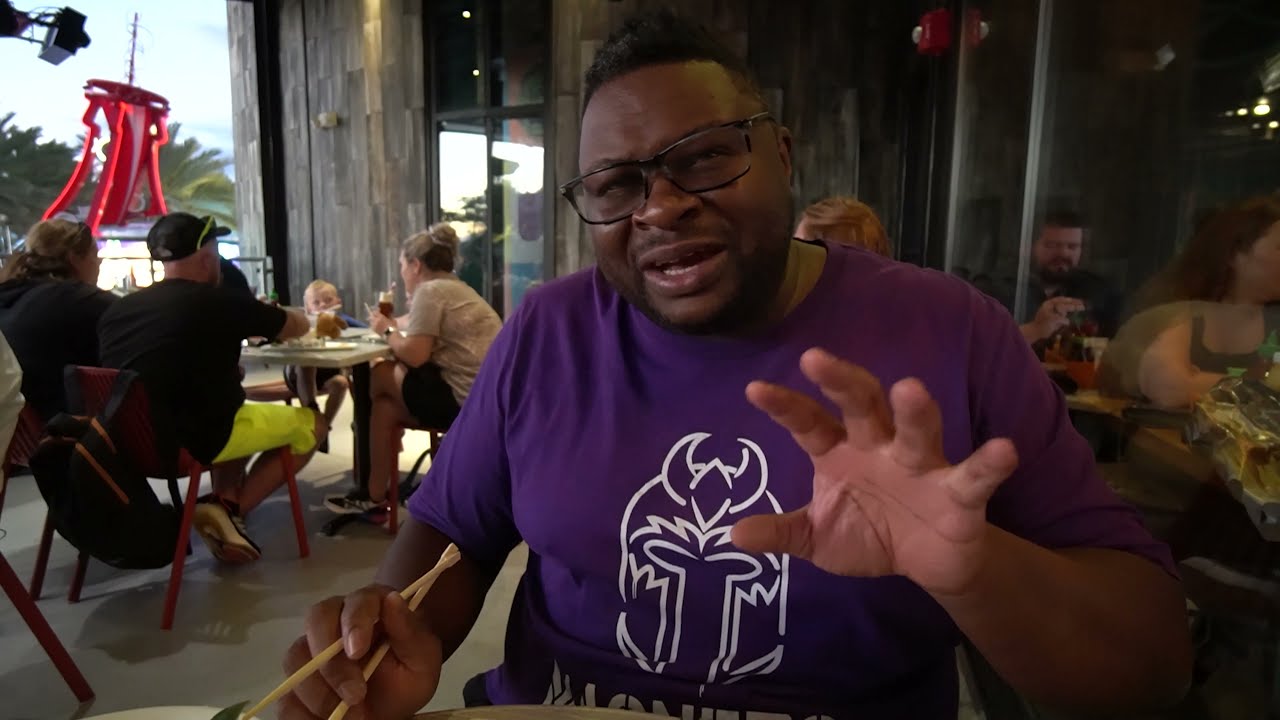In a bustling outdoor restaurant, a black gentleman sits front and center, animatedly engaging with someone off-frame. He wears glasses and a purple T-shirt, adorned with what appears to be an outlined design of a Mandalorian mask or a Viking helmet. His expressive demeanor is highlighted by his left hand, which is outstretched, palm open, and his right hand, which clutches a pair of chopsticks. The setting is vibrant, with a bright sky and trees visible beyond the patio area. Behind him, a mix of patrons are dispersed around low tables; on the left, a group of three to four people are eating and conversing beneath a Chinese streamer hanging in the window, while on the right, near the glass walls of the restaurant, a family sits with a baby in a high chair. The scene captures a lively moment of interaction amidst the warm, inviting atmosphere of the restaurant, characterized by dark brown walls and the reflections of diners in the glass.